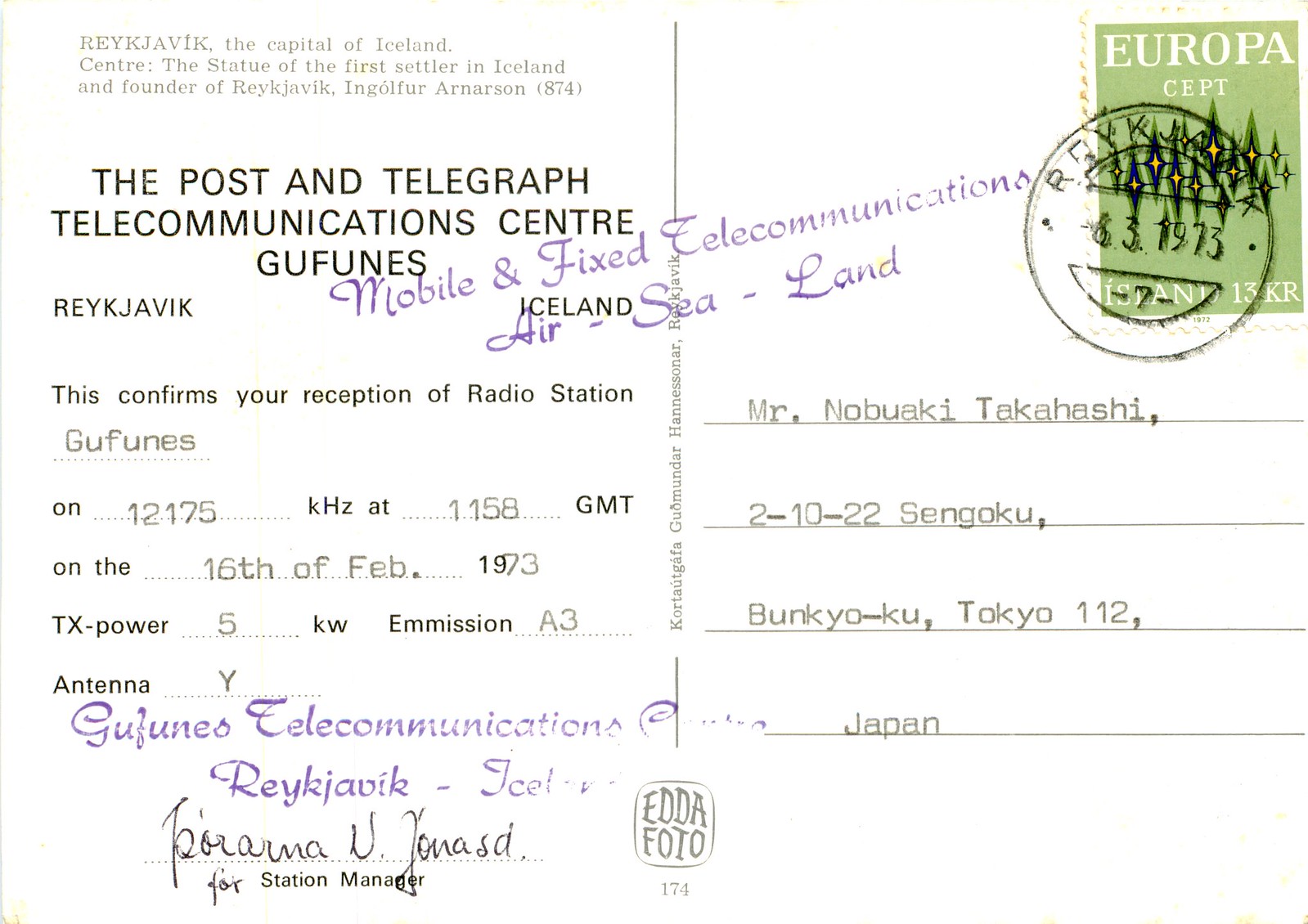The back of an older postcard sent from Reykjavik to Mr. Nobuaki Takahashi in Tokyo, Japan, features several distinctive stamps, including a Europa stamp and one from Reykjavik dated June 3, 1973. The postcard confirms the reception of radio station Gufunes on the frequency 12175 kHz at 1158 GMT on February 16th, 1973, with a transmission power of 5 KW and an A3 emission using antenna Y. The stamp in the top right corner is positioned vertically and is rectangular in shape. Text in purple lettering states, "Mobile and Fixed Telecommunications Air, Sea and Land." Additionally, the top section of the postcard details that Reykjavik, the capital of Iceland, was founded by Ingolfar Arneson in 874. The recipient, Mr. Nobuaki Takahashi’s address, is listed as 2-10 Sengoku, Tokyo, Japan.